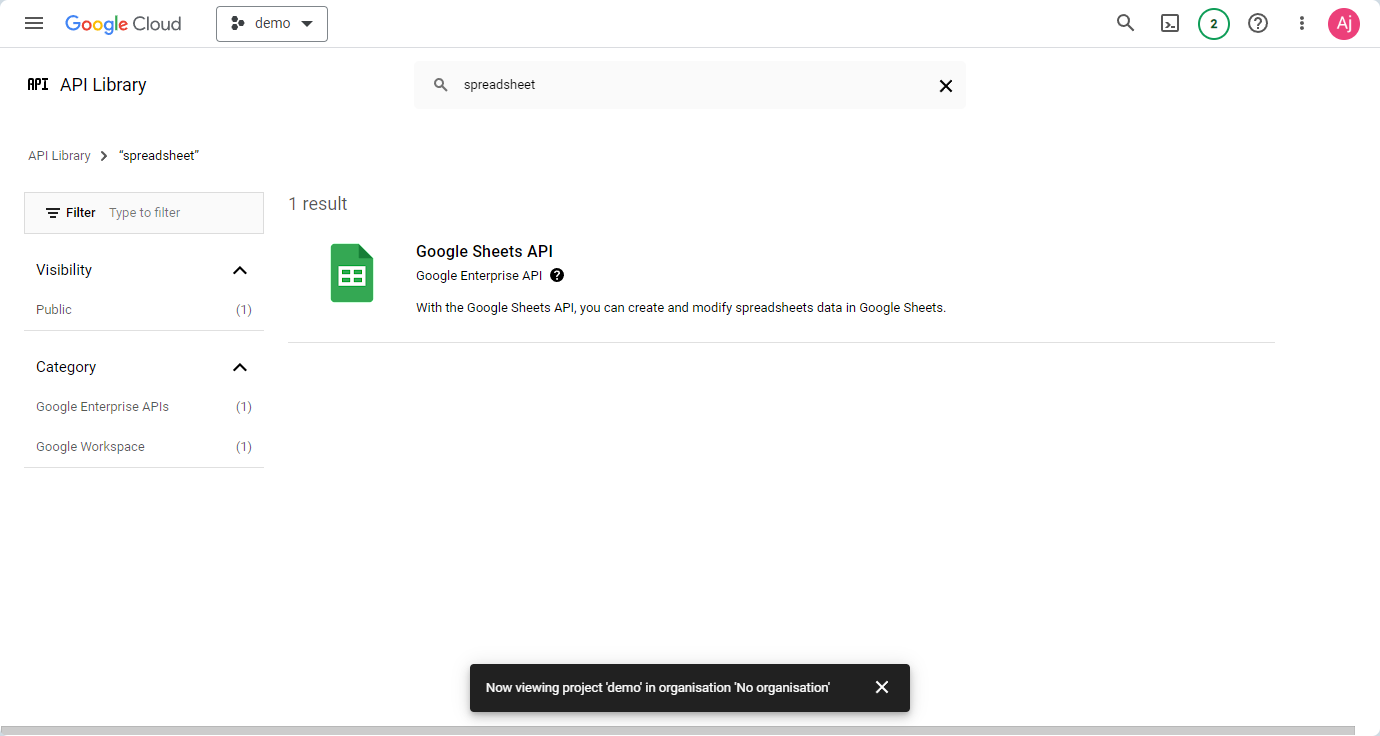This is a detailed screenshot of a demo page on the Google Cloud platform. The background is predominantly white, complemented by black text. On the top left, the distinctive "Google Cloud" branding is present, with "Google" rendered in its trademark vibrant colors: blue, red, yellow, and green.

At the top of the screen, a gray bar spans the width. On the left of this bar are three horizontal lines, indicating a collapsible menu. Adjacent to these lines, the text "Google Cloud" appears. Towards the right, there's a gray box containing a dropdown menu labeled "demo". Further to the right, several icons are visible, including a magnifying glass for search, a question mark within a circle, and a profile circle, among others.

Below this gray bar, on the left-hand side, the text "API library" is displayed prominently. In the main content area, a central gray search bar features a magnifying glass icon. Inside this bar, the term "spreadsheet" is typed, accompanied by a delete "X" option on the far right.

The navigation bar on the left starts with a gray box labeled "filter" and an adjacent prompt "type to filter." Below this section, "visibility" is listed with an upward caret, indicating an expandable menu. Under "visibility," "public (1)" is noted, followed by a dividing line. Continuing down, "category" also features an upward caret, and under this, "Google Enterprise APIs" and "Google Workspace," both list "(1)" results respectively.

One result is displayed for "spreadsheet," showing an icon for Google Spreadsheets. This icon depicts a green document with its top right corner folded and containing four squares. Next to the icon, the text reads "Google Sheets API," followed by "Google Enterprise API" and a clickable question mark for additional information. Below, a description states: "With the Google Sheets API, you can create and modify spreadsheet data in Google Sheets."

At the very bottom center of the screen is a prominent black bar with the text "Now viewing project demo in organization: no organization." Below this text is a thin gray line running the width of the screen.